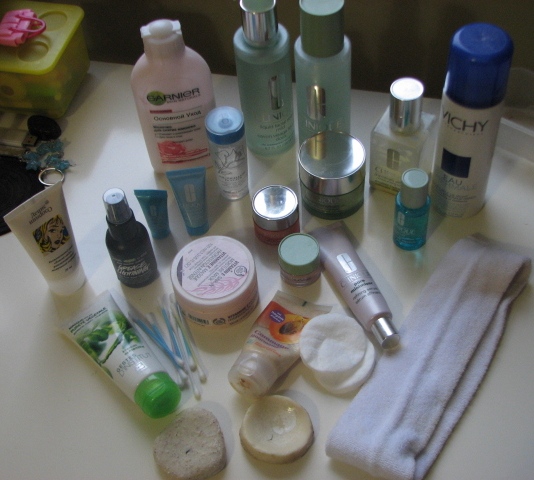This overhead photograph captures a section of a bathroom countertop, showcasing an array of self-care items neatly arranged. The off-white countertop hosts a variety of containers, varying in size and shape. Among the items are makeup applicators and removers, and a hairband likely used for keeping hair back during routines.

Prominently featured is a pink Garnier bottle, presumably conditioner, flanked by two matching green bottles from Vichy. There is also a bottle that appears to be cologne, adding to the mix of different products. The diverse collection displays a spectrum of colors, including green, pink, purple, and light blue, all standing in contrast to the subdued countertop.

Some containers are traditional with dispensers on top, while others are travel-sized and positioned on their lids. The photograph captures approximately 20 to 30 items, though the edges hint at additional objects just out of view. The image is well-lit, though slightly dim, offering a clear yet gentle look at this curated assortment of personal care essentials.